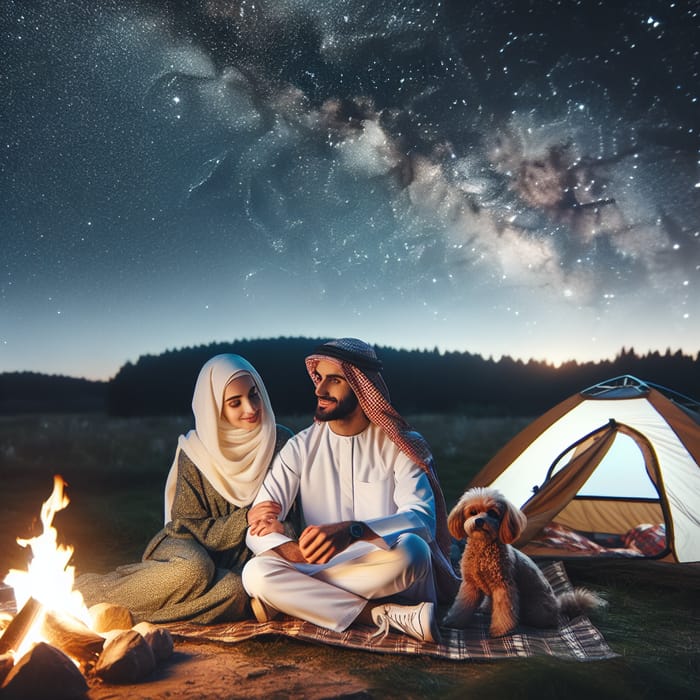The image depicts a young couple camping in the countryside, sitting in front of a generous campfire bordered by rocks. They are seated on a red and white plaid picnic blanket. The couple, who appear to be Middle Eastern, are dressed in traditional attire; the woman is wearing a white hijab and a brown outfit, while the man is dressed in white with a red head covering that has a long flowing cape-like structure. The woman wraps her arms around the man’s arm as he looks into the distance, and she gazes downward. Next to the man is a small fluffy dog, which looks like a poodle, attentively looking forward. Behind them stands a small compact tent, brown on the sides with a white front and brown door. The tent’s door is open, revealing sleeping bags inside. The scene is set on patchy ground, and in the background, a forest and expansive land stretch beneath a night sky scattered with stars and a few clouds, accentuating the remote, serene environment.